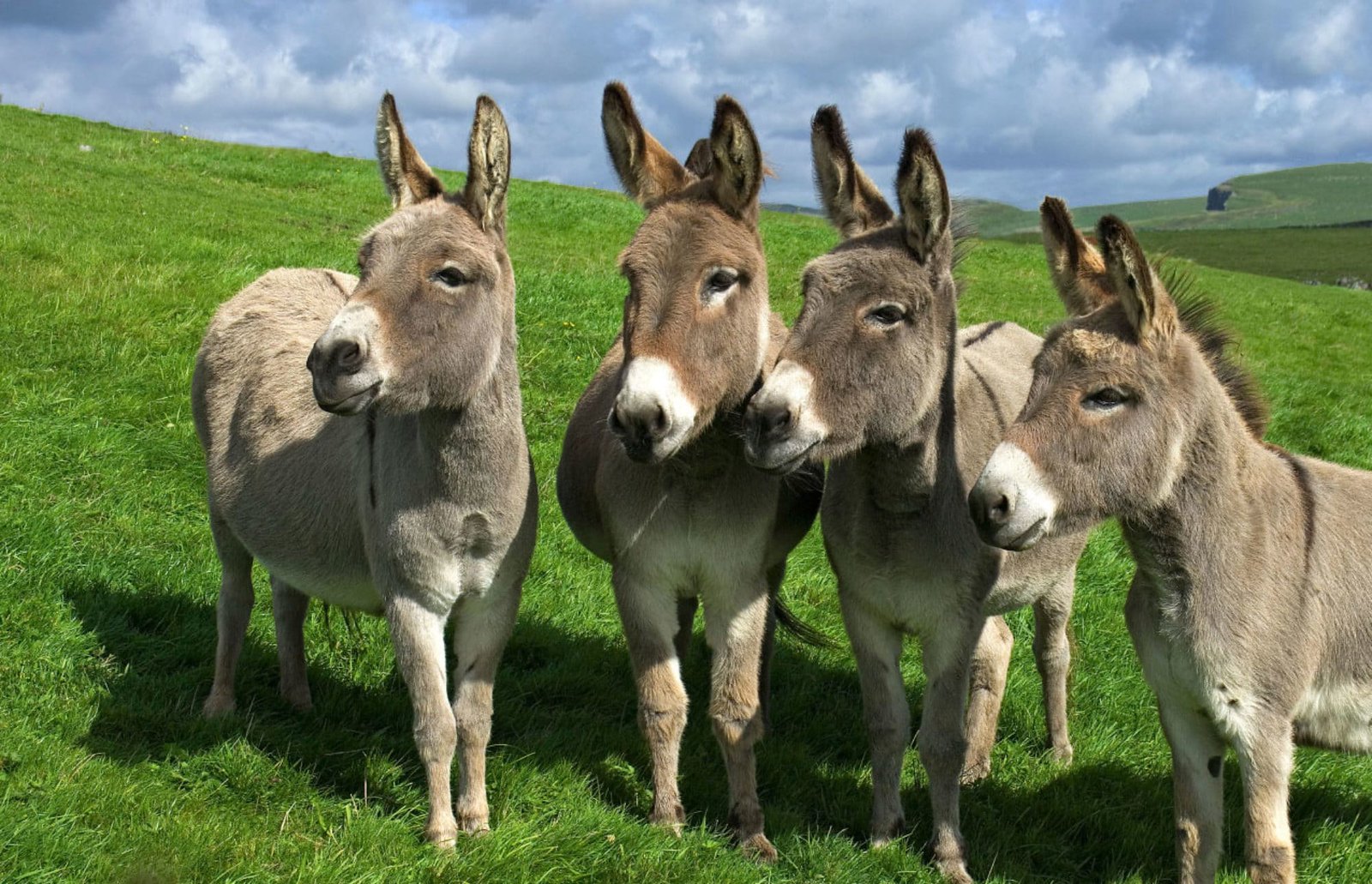This photograph captures four donkeys, also referred to as burros, gathered on a lush, green grassy hillside on a partly cloudy day. The donkeys, with varying shades of tan to light and dark brown coats, are standing closely side by side, slightly fanned out with their heads aligned and hind legs splayed behind them. Each donkey has distinct pointy ears that stand upright and a white spot on their snouts, along with a light brown chest. They all have dark brown manes and dark eyes that seem to squint slightly due to the sunlight. These donkeys are gazing intently off to the left, appearing to focus on the same distant point. The background reveals rolling green hills that stretch far into the countryside, with a mountain top visible against a sky dotted with thick, low-hanging clouds, indicating a serene but expansive rural setting, far removed from urban areas.